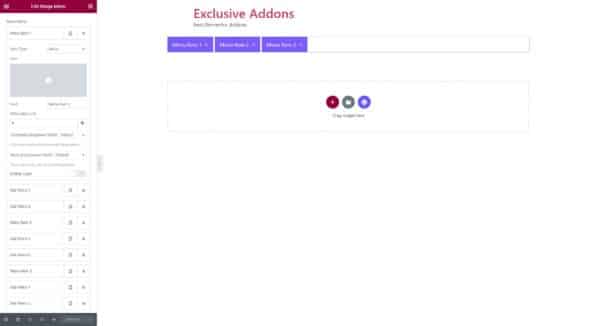The image depicts a white page with a distinct header that reads "Exclusive Add-ons" in red print, prominently centered towards the top. Below the header, there is a block of black text, although it is too blurry to decipher. Following this text, the layout features three blue rectangles aligned horizontally, each with white text in their centers, which is also unreadable. Beneath these rectangles is a long white horizontal rectangle.

Further down the page, there is a larger rectangle outlined with a thin gray line. Inside this rectangle are three circles, each circle containing a unique color and a specific icon in its center. Below these circles, there is more text, but it is blurry and illegible.

On the left side of the page, there is a vertically-oriented menu. The top of the menu features a red bar, while the bottom is marked by a dark gray bar. In between, the menu contains several smaller boxes with text that is too blurry to read, and a larger gray box positioned towards the top of the menu.